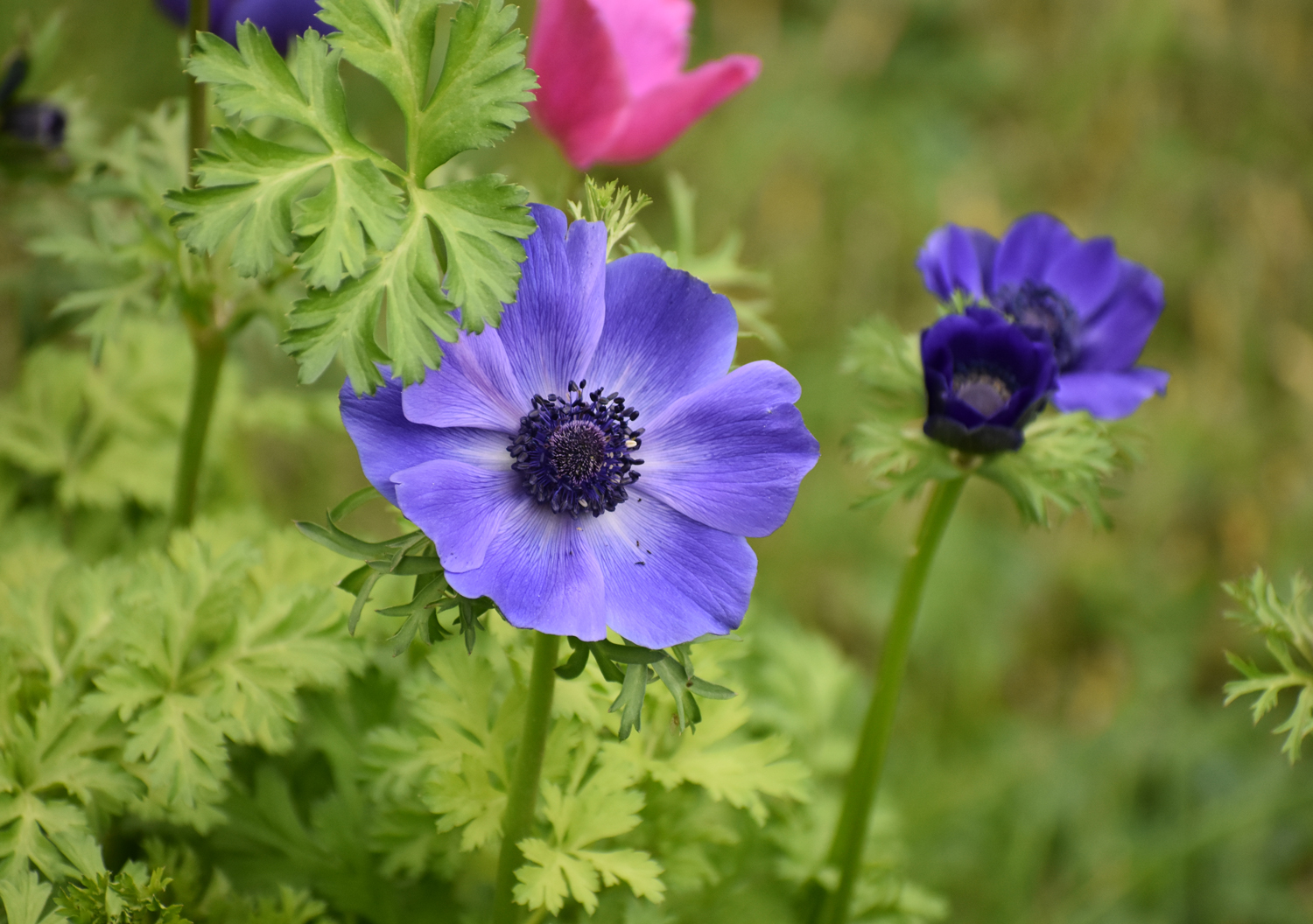In this detailed and vibrant outdoor nature photograph, we zoom in on a captivating scene dominated by tall, delicate purple-petaled flowers. Each flower boasts about 10 petals that transition from a lighter shade near the dark purple stamen at the center, to a richer, darker purple hue at the outer edges. The petals exhibit a slight ripply texture, enhancing their delicate appearance. The central focus is a large purple flower standing prominently on a green stem, surrounded by bright green, parsley-like leaves that add a lush backdrop to the composition.

To the right, another purple flower bends gracefully to the side, though it appears more blurred and indistinct, hinting at its position further in the background. Above the central purple flower, a pink tulip-like bloom is faintly visible, but also blurred, indicating its distance from the main subject. The left side of the image teems with bright green leaves growing upwards, though they lack blooming flowers. Notably, the photograph incorporates a subtly blurred effect, especially on the right side, lending a dreamlike quality to the scene and emphasizing the vivid, sharp focus on the central purple flower.